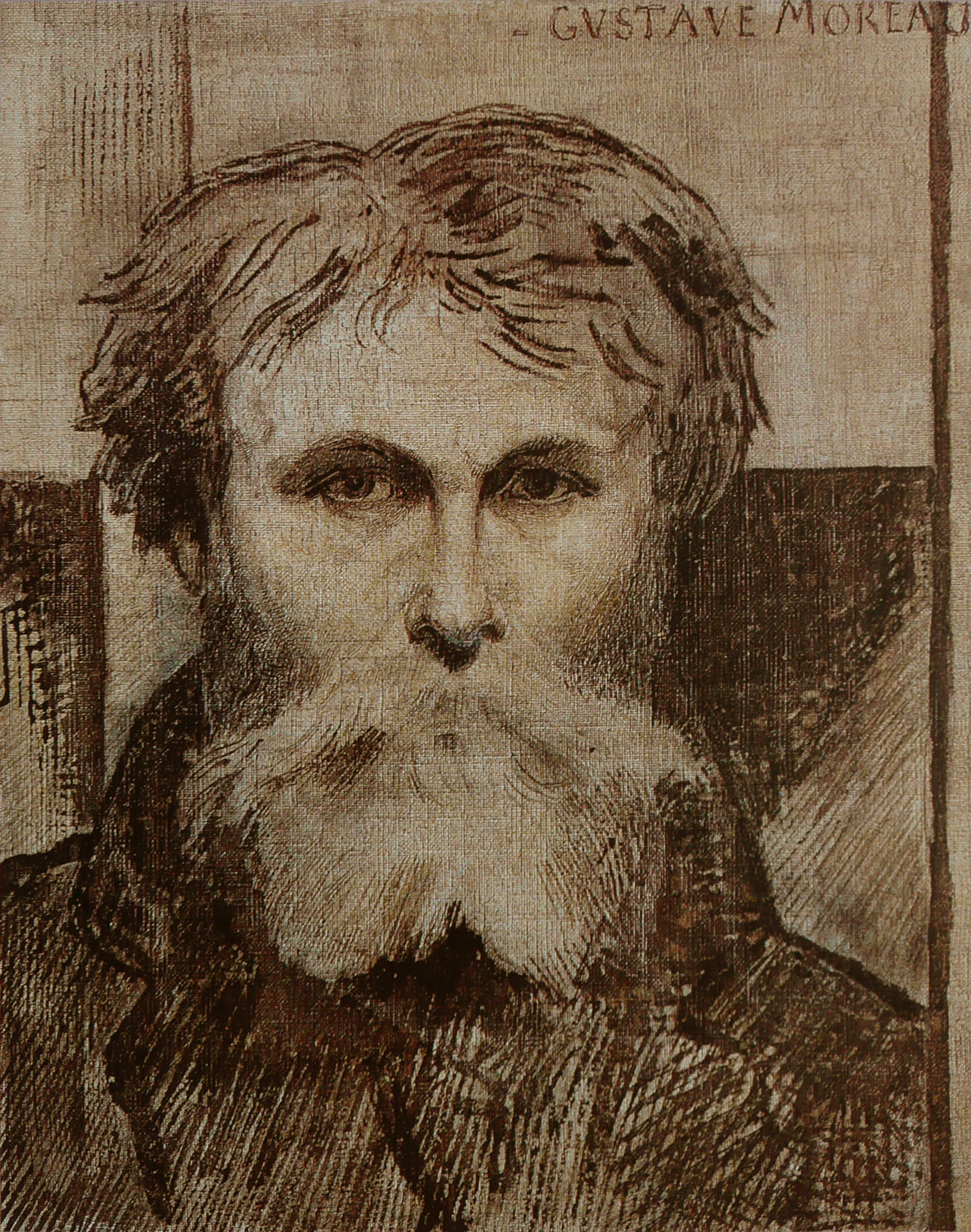This image depicts a muted ink or pencil drawing, rendered in black, brown, and beige tones, on a textured, brownish-tan paper. The artwork features a man from the chest up, with the signature "Gustave Moreau" at the top. The man has wild, bushy hair that falls just past his ears and is slightly parted on the left. His expressive eyes, soft and brown, gaze directly at the viewer, set beneath thick, brushy eyebrows. He sports a full, brushy mustache and a medium-sized beard covering his mouth and jawline, giving him a rugged appearance. His facial features include a long, pointed nose. The man is dressed in a heavy, dark overcoat with a high collar that reaches up to the base of his ears, suggesting he might be outdoors. The background is more of a line drawing, non-definable, and evokes a dark, somewhat somber mood, complementing the overall aesthetic of the piece.